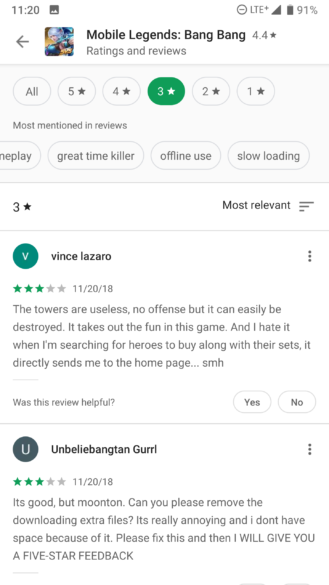A user is depicted browsing the Google Play Store, specifically viewing the game "Mobile Legends: Bang Bang," which holds a rating of 4.4 out of 5 stars. The screen shows that the user is in the process of rating the app, potentially considering giving it 3 stars. Displayed tags indicate common review themes such as "great time killer," "offline use," and "slow loading." Below, several 3-star reviews are visible, suggesting filtered results based on ratings. One review criticizes the game's towers, calling them "useless" and easily destroyed, adding that it diminishes the fun. The reviewer also expresses frustration with the navigation, which redirects them to the homepage when trying to purchase heroes and their sets. Another review acknowledges the game's positives but pleads with the developers, Moonton, to remove the requirement for downloading extra files, citing limited storage space. Both reviews were posted on the same day in November 2018, possibly marking the game's release date. The interface features a generally dark background with black text, and there are sorting options by relevance or date.